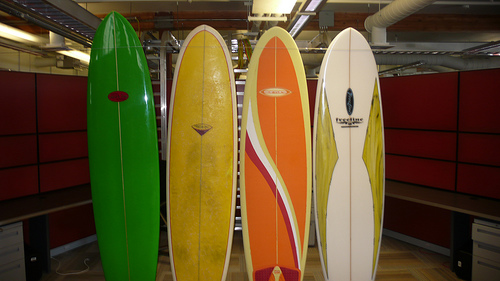This is a photo taken with an average camera, capturing four surfboards standing upright in semi-focus against a dark background. The image is set indoors, likely in a warehouse or a storage unit characterized by red-colored walls, overhead fluorescent lighting, and possibly some cubicles in the backdrop. Each surfboard varies in color and design: the leftmost is a shiny green and slightly taller than the other three, the second one is predominantly yellow, followed by an orange one with yellow and white accents and a swoosh design in the middle, and the rightmost surfboard is mostly white with a yellowish design in the center that appears somewhat older and dingier. Although the surfboards display various logos, the logos are too small to read. The bottom part of the image is cut off, suggesting the boards are either propped up by unseen slats or hanging, though no visible supports like ropes or twine are evident.